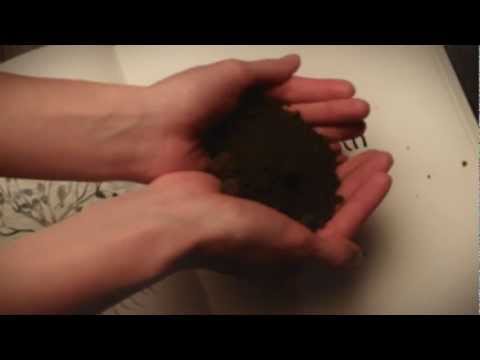A horizontal rectangular photograph features a pair of fair-skinned hands, likely a woman's, cupped together and holding a mound of dark brown or black dirt. The hands, extending from the left side of the image and visible up to the wrists, are centrally positioned. The background consists of an open book with white pages, lying on what appears to be a dark surface. On the left page of the book, there's a black and white illustration of a tree, while the right page has some text obscured by the hands. The image is framed with black letterboxing at the top and bottom, further emphasizing the central subject. Small specks of dirt are scattered around, adding to the detailed texture of the scene. The overall color palette includes shades of brown, peach, olive, white, and black, suggesting a domestic setting, possibly in a house or bedroom.